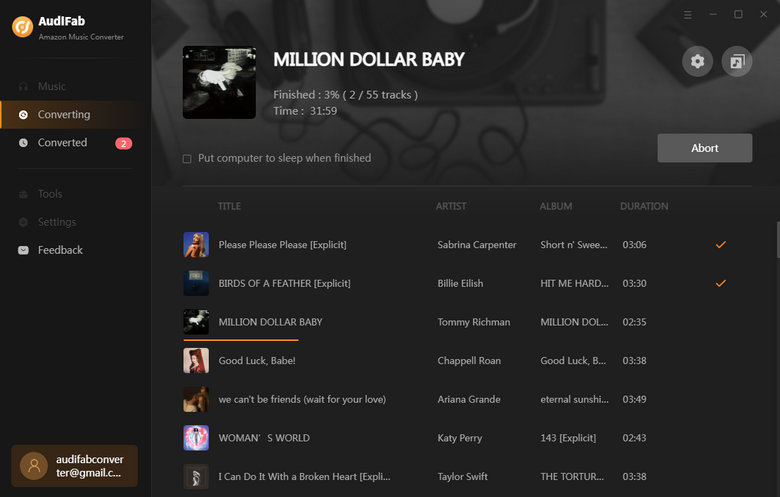The image displays the interface of an audio or music-playing site named "Audifab," indicated by the white text in the top left corner. Adjacent to this text is a circular logo with an orange background and white shapes.

The interface comprises four main sections listed vertically on the left side. The first section, "Home," is grayed out, indicating it is not currently selected. The second section, "Converting," is highlighted, signifying it is the active tab. Below this is the "Converted" section, marked with a small red oval to the right. The final section is labeled "Tools."

In the bottom left corner, a user's email is displayed. Directly above the email is the word "Feedback," accompanied by an envelope icon. Above "Feedback" is "Settings," denoted by a gear icon.

The center top of the interface features the name of an album, "Made You Look." To the left of this title is a square image depicting two women against a pink background.

Below the album details, several song titles are listed: "Baby Don't Hurt Me," "Chemical," "Mine," "The Other Point of View," "Eyes Closed," "Made You Look," and "Cooped Up / Return of the Mac."